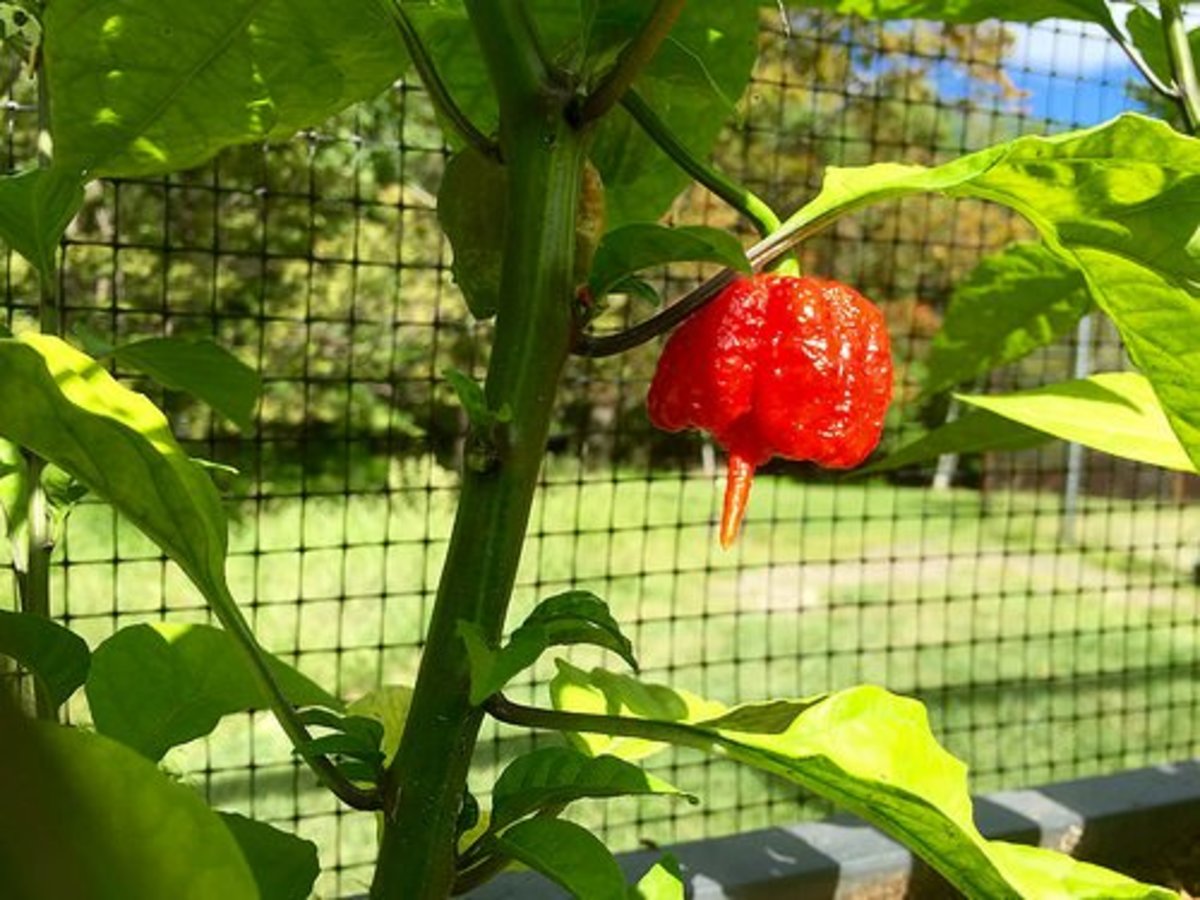The photograph taken during the day features a vividly detailed scene of a garden plant, focusing on a large, shiny, and somewhat glossy red fruit or vegetable that resembles a bell pepper. It hangs from a green stem with vibrant, fresh green leaves, highlighted by sunlight. The red item has an almost wrinkled texture and has a small spike or protrusion coming from its center. Behind this plant is a mesh fence with square-shaped holes that serves to protect the garden. The fence has a gray rim at the bottom, encasing rich brown soil in a container. In the top right corner of the image, a small glimpse of blue sky with a white cloud is visible.